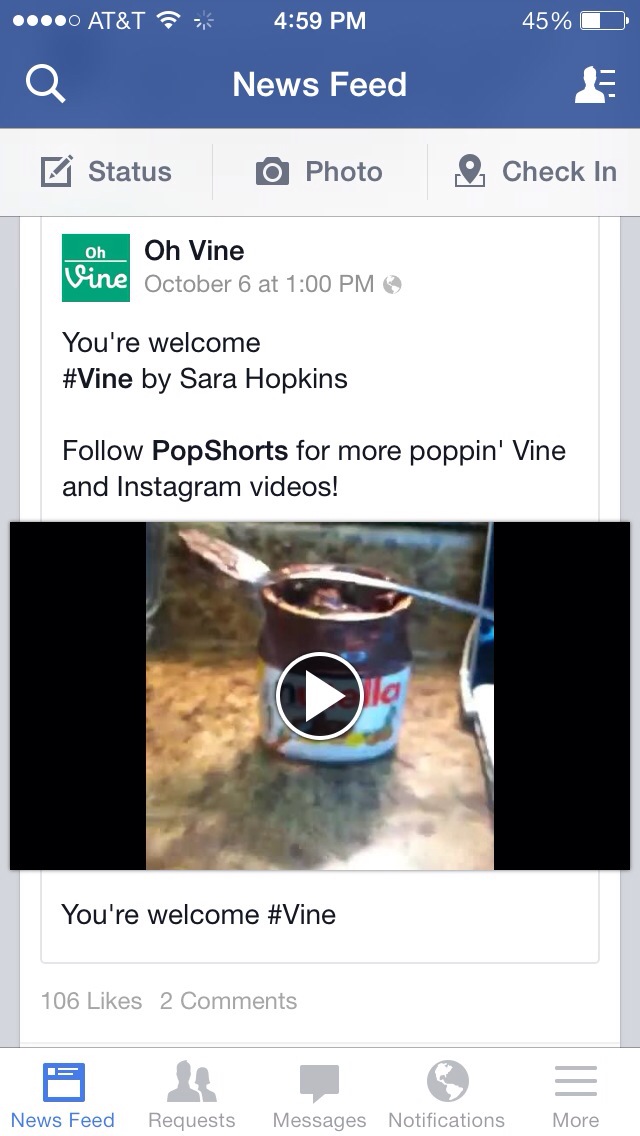This detailed caption provides a comprehensive description of the screenshot, incorporating all the shared and repeated elements from the three provided captions:

---

This screenshot captures a Facebook news feed displayed on a mobile phone. At the top of the image, a blue horizontal bar features the AT&T carrier signal with four out of five bars, the time reading 4:59 p.m., and a battery indicator showing 45% remaining. Beneath the blue bar, there are options for 'Status,' 'Photo,' and 'Check-in,' along with a magnifying glass icon for search.

The main content of the post is from an organization named O-Vine, dated October 6th at 1 p.m. The post includes a message saying, "You're welcome, #Vine by Sarah Hopkins. Follow Pop Shorts for more Pop and Vine and Instagram videos." The central focus of the screenshot is a paused video of an open Nutella jar with a spoon resting on top, coated with some Nutella, indicating it has been dipped and used.

This post has garnered 106 likes and 2 comments. At the bottom of the screen, navigation options include 'News Feed,' 'Requests,' 'Messages,' 'Notifications,' and 'More,' each represented by distinct icons, including a world icon for Notifications and three vertical lines for More.

---

This caption efficiently consolidates the details, offering a vivid and accurate description of the screenshot.